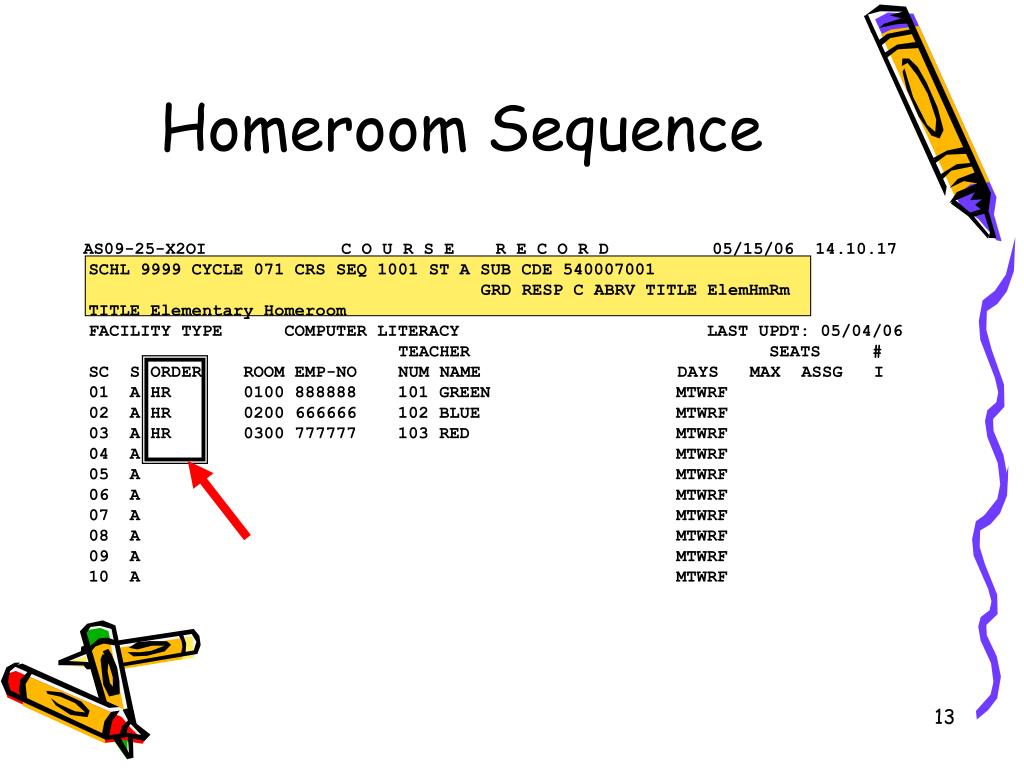The image depicts a cartoonish, computer-generated table titled "Homeroom Sequence," set on a white background. In the upper right corner, there is a purple crayon with a yellow label and a squiggly purple line extending from the top right to the bottom right. The number 13 is also located in the bottom right. The table itself is a detailed spreadsheet with various columns and rows, featuring course records, facility types, and teacher assignments. Key entries include "AS09-25-X2OI," "Course Record 515.06.14.10.17," and "SCHL-9999-071-CRS-SEQ-1001-STA-SUB-CDE-54007001" in a yellow banner, followed by "Title Elementary Homeroom," and "GRD RESP C ABRV TITLE HMRM." The left column lists "SC" followed by numbers 01 to 10. Adjacent columns detail "Order HR HR HR," Room numbers "0100, 0200, 0300," and "Teacher NUM 101-103" with names corresponding to colors—Green, Blue, and Red. Days of the week are listed as "MTWRF" in a repeated column. Another column labeled "Seats" includes "MAX ASSG" entries. The bottom left of the image features three more cartoon crayons—one red, one green, and one yellow—each with a classic Crayola-style yellow wrapping.